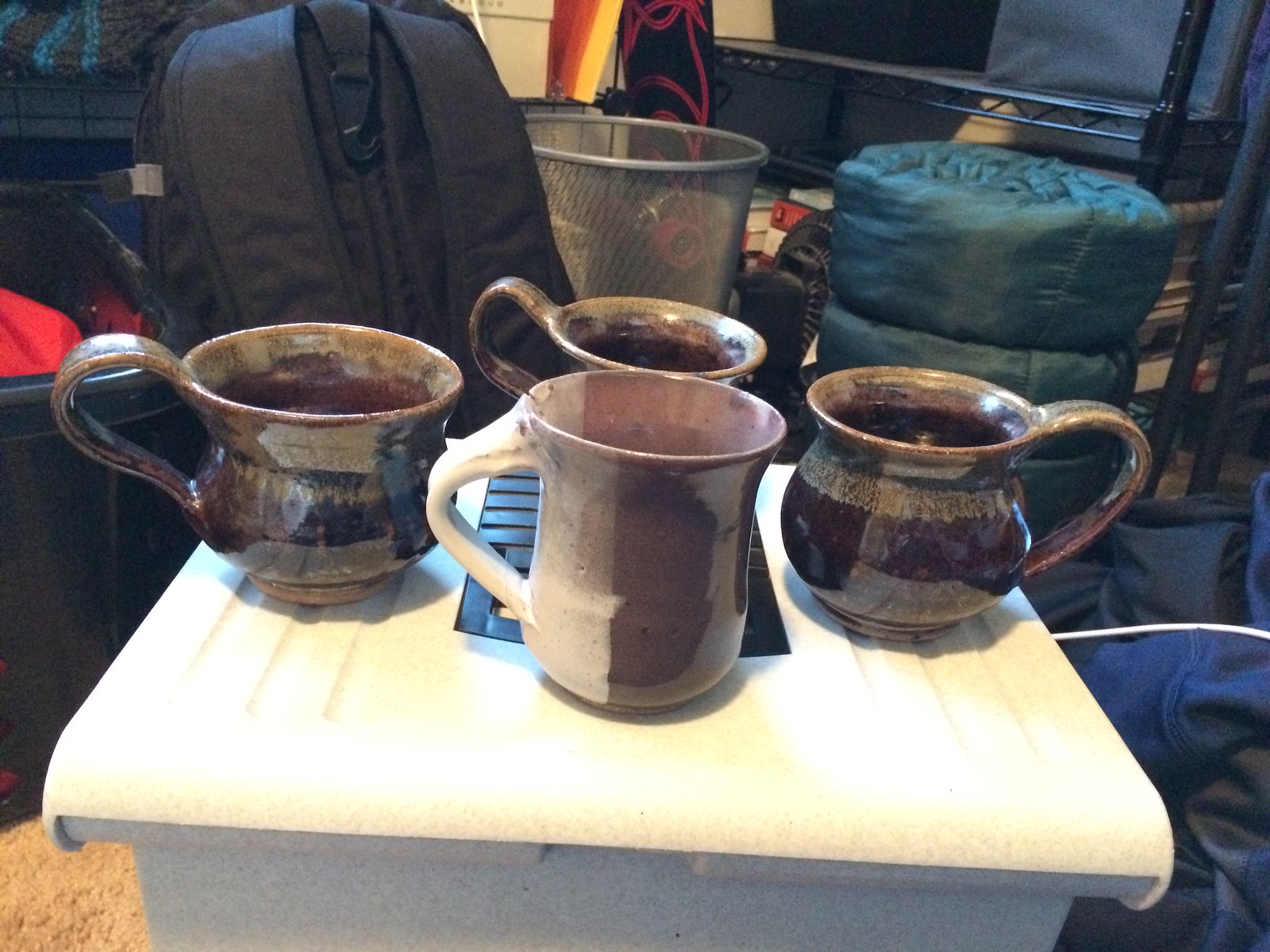In a cluttered room filled with various items, a makeshift table, possibly a white container with a lid, serves as the central focus. On top of this surface, there are four large, uniquely designed coffee mugs. The front-most mug features a distinctive white and reddish-brown color scheme and stands taller but narrower than the others. The remaining three mugs, nestled behind, share a common bronze and black palette with slightly different shapes and patterns, all adorned with large, uniquely curved handles. Surrounding the makeshift table, the room is strewn with a variety of belongings, including a black backpack, a rolled-up old sleeping bag, a wire trash can, and a stack of metal shelves. Additional details in the scene include a jacket, a possible crocheted item in the top left, a skateboard hanging behind the trash can, boxes, and books stacked on the wire shelf, as well as piles of clothes, contributing to the overall impression of a cluttered personal space.